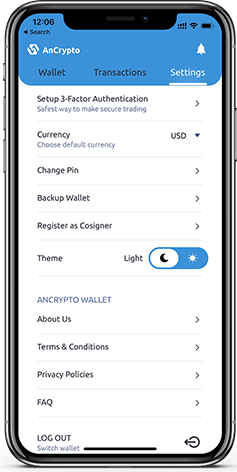Caption: 

A detailed screenshot of the AnCrypto mobile app settings tab. The top of the screen features a light blue header with the AnCrypto logo and name prominently displayed. Below the header, the settings options are listed on a clean white background. The available selections include setting up three-factor authentication, changing the currency display, changing the PIN, backing up the wallet, and registering as a cosigner. Users can also choose between light and dark themes for the app interface. Additional options include accessing the 'About Us' section, reviewing terms and conditions, privacy policies, FAQs, and logging out. The power off, switch wallet, and logout options are located at both the bottom and bottom-right corner of the screen. A reminder notification icon is visible at the top right-hand side. The overall layout is user-friendly and straightforward, capturing a general view of the application’s settings page in action.